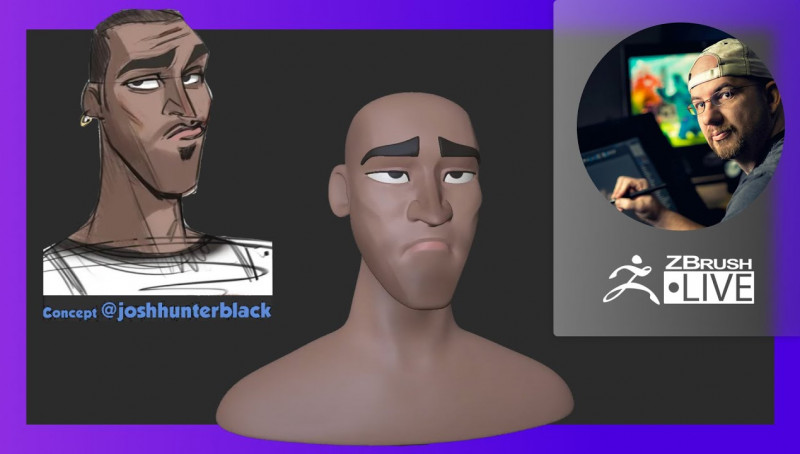This image showcases an intricate design concept for a website or logo, featuring two distinct characters. On the left, a hand-drawn sketch lays the foundation, while on the right, a highly detailed 3D model brings the character to life. The original concept was created by George Hunter Black, highlighting his unique artistic vision. To the right of the characters, a circular logo featuring a human figure prominently displays the text "ZBrush Life." The color palette in this composition primarily includes rich purples, blacks, and blues, accented by touches of white, gray, and brown, creating a visually cohesive and striking design.